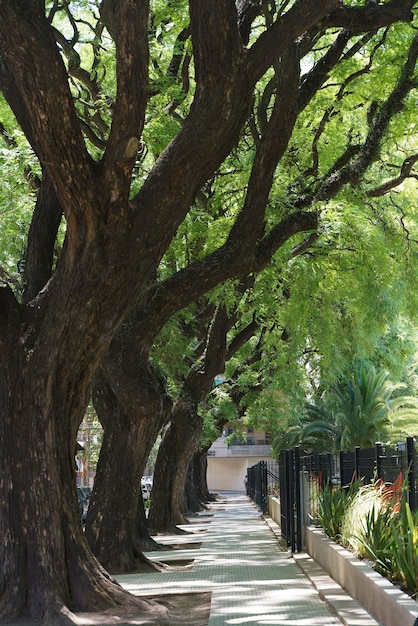This color photograph captures a serene outdoor scene of a tree-lined concrete pathway, resembling a sidewalk with a grid-like pattern. Prominently on the left side, there are multiple thick, dark brown tree trunks with extensive branches that spread across the top portion of the image, creating a natural canopy. The branches are adorned with thin, light green leaves, indicative of springtime. Four trees are lined up closely behind each other, adding depth to the scene. To the right, a black wrought iron fence runs alongside the path, extending all the way to the center of the background. Adjacent to the fence, there is a raised planter bed containing tall, green grassy plants and what appear to be orange-red tulips. The shadows of the trees cast intricate patterns on the concrete below, enhancing the tranquil ambiance of the path.